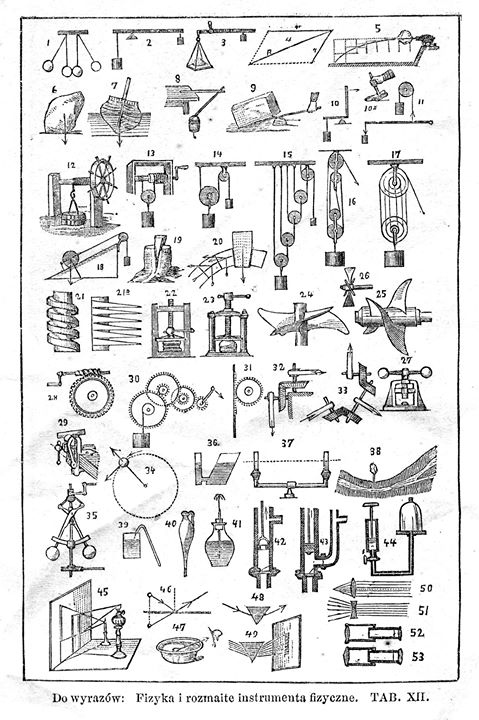This vertical-rectangular, black-and-white image features a detailed, printed illustration of various scientific and mechanical tools, numbered 1 through 53. The illustration includes several sets of pulleys, levers, weights, pistons, gears, and vices, each meticulously drawn to depict its function and design. The top row showcases pendulums, followed by levers, pulleys, and then an array of weight-moving items. Below these, there are additional mechanical parts such as vices and gears. The tools are arranged systematically, with descriptions written underneath in a foreign language, possibly Polish. The image is bordered in black, with the details and text maintained in stark contrast against a white background.